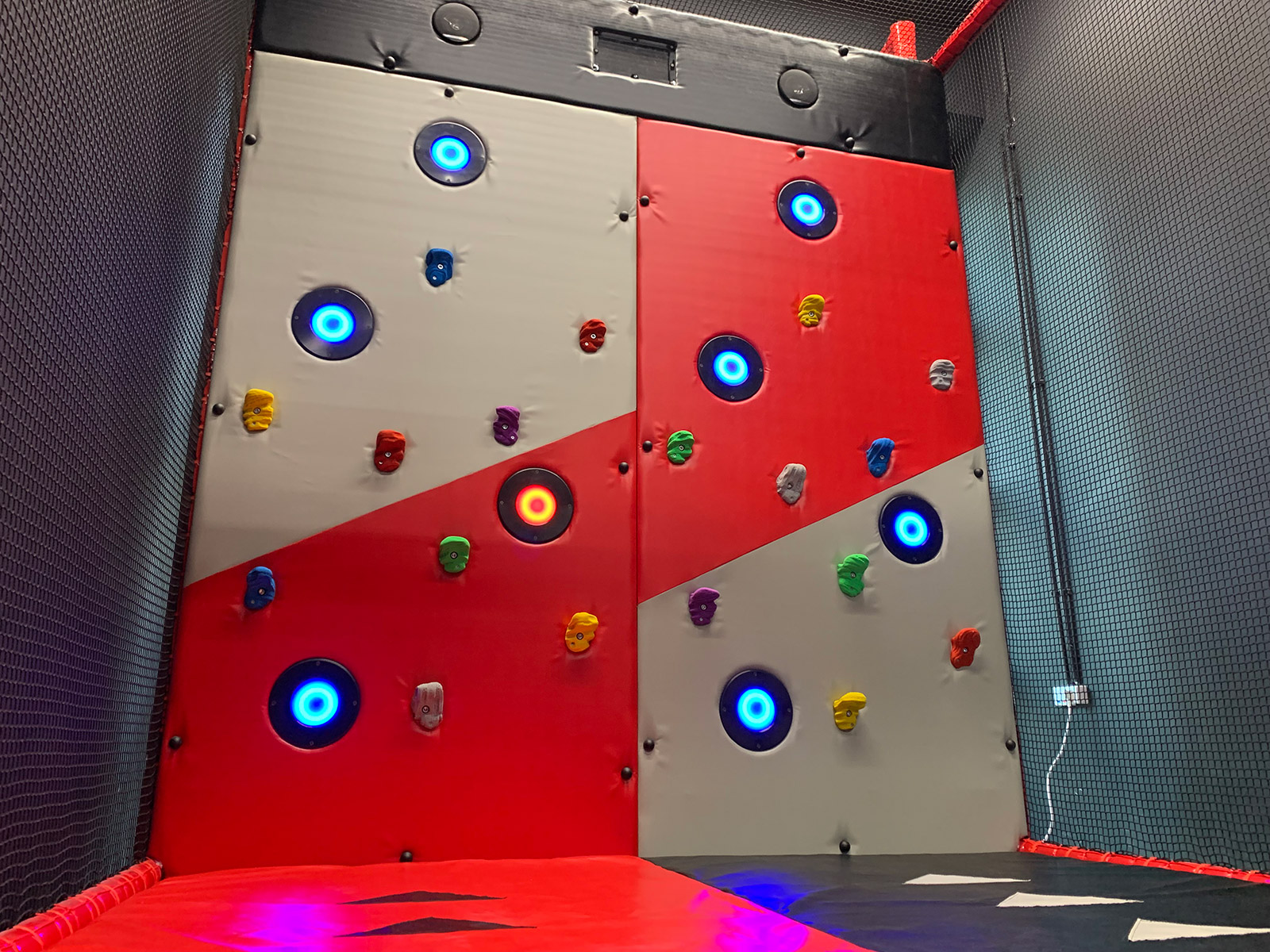The image depicts a digital and futuristic rock climbing wall situated in what appears to be a gymnastics or trampoline play center. The wall features traditional multicolored climbing grips in yellow, red, green, purple, blue, and brown, secured onto a black, gray, and red padded surface. Additionally, the wall sports illuminated circles—primarily blue with one red circle—suggesting a game element where climbers aim to touch the blue circles while avoiding or interacting differently with the red one. The climbing area is bordered by netting on both sides, and the floor is covered in padded mats in red, black, and beige. There are also black and white directional arrows on the floor indicating the ascent route. A plug attached to the wall hints at the digital nature of the climbing setup.